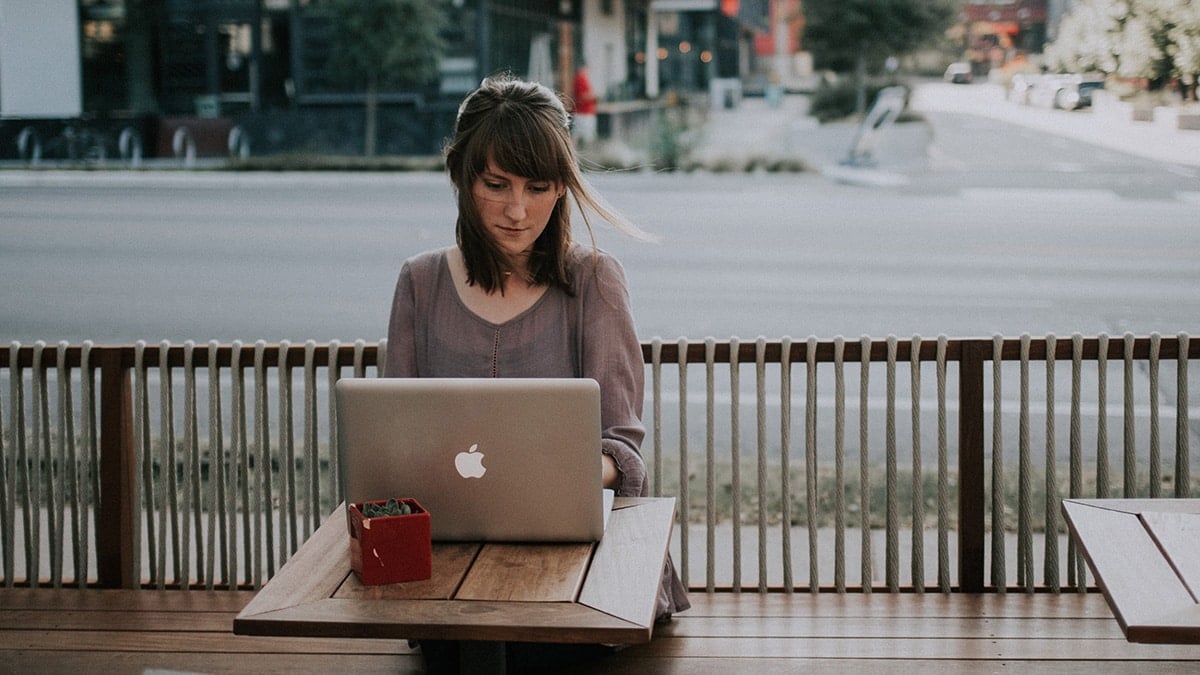In this detailed color photograph, a woman in her 30s is intently working on an Apple laptop while seated on an outdoor patio. The woman has shoulder-length dark brown hair, with bangs and some strands being gently blown by the breeze. She is dressed in a long-sleeved gray blouse and is sitting at a small, square wooden table that is barely large enough to hold her laptop and a small red planter with a green plant. Behind her is a waist-high wooden railing and a street with various buildings that are out of focus. The street runs both vertically and horizontally in the background. The overall arrangement suggests that the woman is engaged in focused office work rather than dining, highlighted against the urban backdrop devoid of other people.